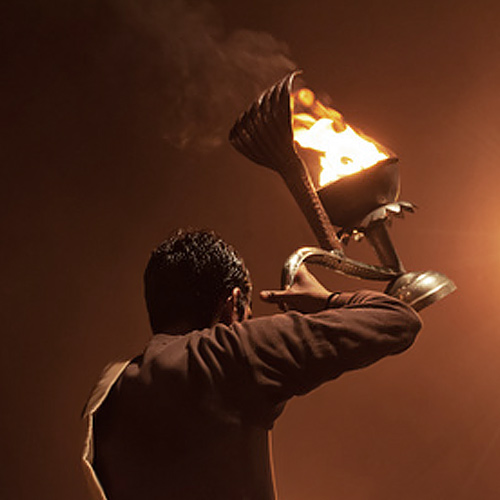In this photograph, an evocative scene from a movie is captured in rich chocolate brown tones. A man with short brown hair and tan skin stands at the center, his back partially turned to the viewer. Clad in a brown long-sleeved shirt, he is grasping an intricate brass artifact shaped like a King Cobra with its hood expanded. This impressive object appears to merge a staff with a lamp or lantern, featuring a large, curved handle and an additional arched arm that hovers over the flames. The base of the artifact is round with scalloped edges, and a lid is poised to close over the fire. Smoke curls upward, adding to the mysterious and dramatic ambiance of the dimly lit room.